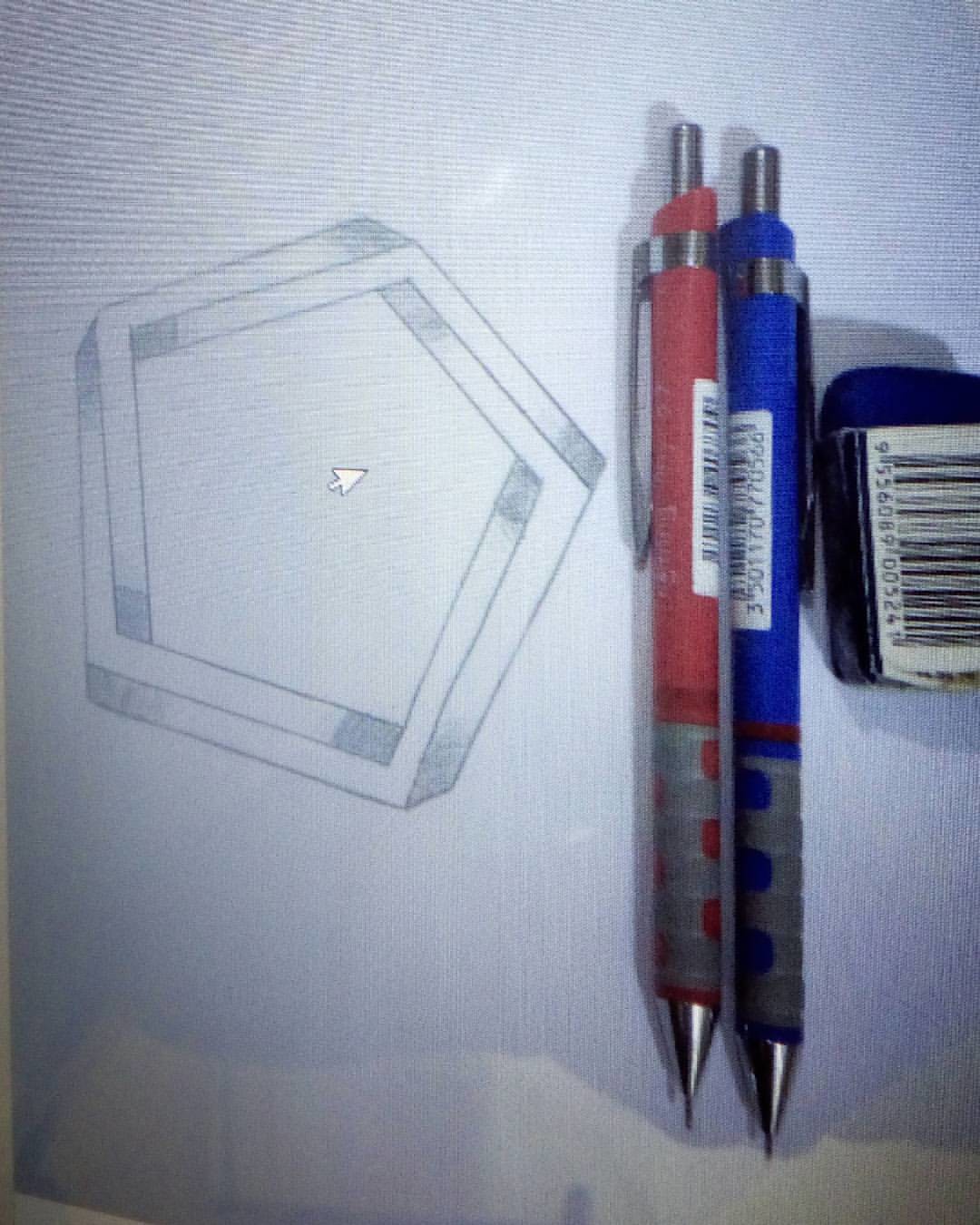The photograph captures a computer screen displaying an image of a neatly arranged composition featuring stationery items and a geometric drawing. Due to the nature of photographing a screen, there is noticeable distortion with crisscrossing lines creating a textured effect across the image. Central to the image is a floating computer cursor. 

On the right side of the displayed photograph, two mechanical pencils are positioned vertically, side by side; the left pencil is red and the right is blue, both featuring gray tops and barcode stickers facing upwards. Adjacent to the right of the pencils is a small dark blue pencil sharpener covered predominantly by a large barcode sticker.

Occupying the left half of the image is a meticulously sketched geometric drawing, done in simple graphite pencil. This drawing features an abstract three-dimensional shape, resembling an intertwining hexagon or octagon. The interwoven bars of the shape are shaded to enhance the 3D illusion, with light rectangles at their edges, creating a dynamic play of perspective within the sketch.